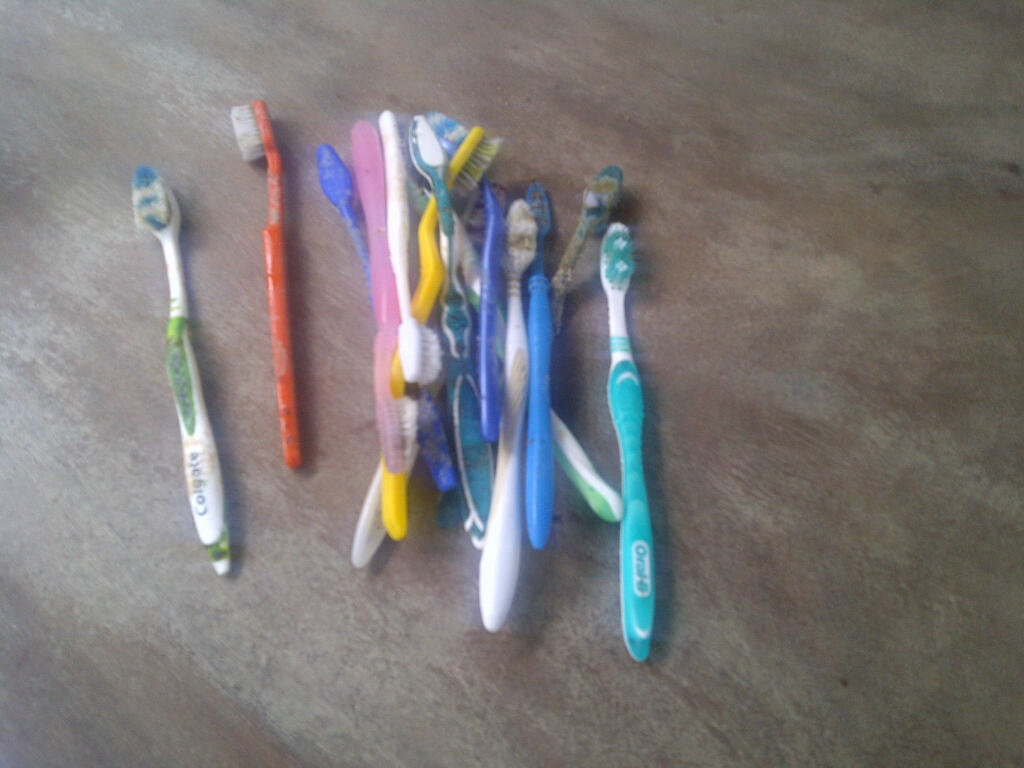This photograph, likely taken indoors and viewed from above in landscape orientation, captures a scene of approximately a dozen used toothbrushes scattered across a grayish-brown, faux-stone countertop. The toothbrushes are a mixture of children's and adult's, featuring a variety of vibrant colors such as blue, yellow, pink, orange, turquoise, and green. Some toothbrushes exhibit two-tone designs with colorful bristles matching their handles. Notably, there is a green and white Colgate toothbrush and a turquoise Oral-B toothbrush among them. The toothbrushes appear dirty and are haphazardly piled together, with a few — including a green and white one and an orangey-red one — isolated to the left, and a turquoise toothbrush standing alone to the right. The photograph is not of high quality, with a blurry resolution, creating an overall impression of a chaotic and unartistic collection of personal hygiene items.